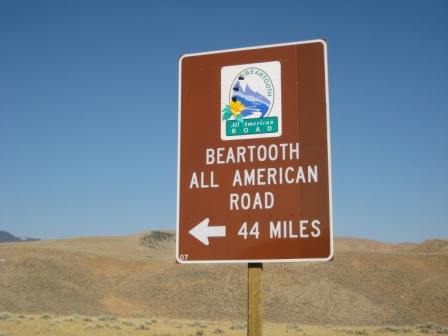The image captures a brown road sign with white text, prominently stating "Beartooth All-American Road, 44 miles" with an arrow pointing left. The sign is mounted on a slender, square wooden post. Above the text, there's a logo featuring a yellow flower with green leaves and a depiction of a mountain range. The landscape behind the sign is a flat, arid desert with sparse shrubs and gradually rising ridges in the background. The sky above is a vivid, clear blue, further highlighting the stark beauty of the desert environment. The scene evokes a sense of adventure and the anticipation of a scenic drive.